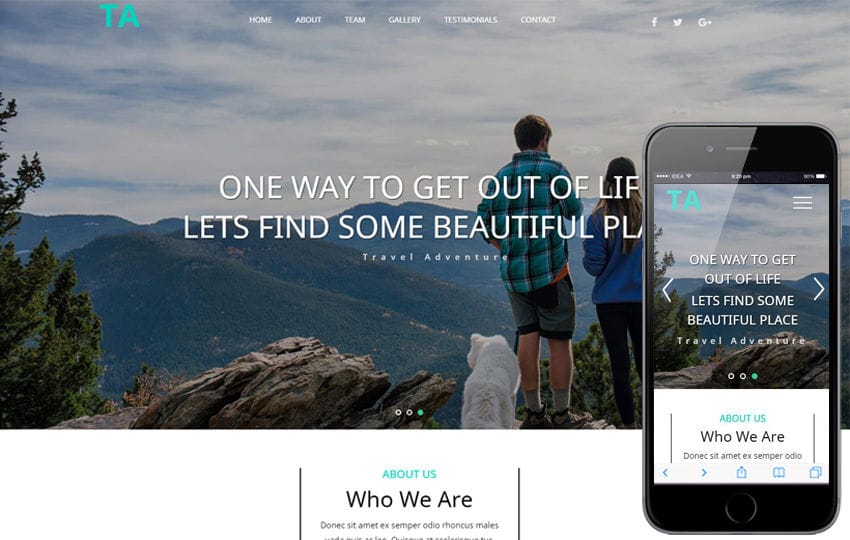The web page features a title "T.A." in teal typography on the left-hand side. The background image showcases a couple accompanied by their white, fluffy dog, standing atop a mountain and gazing over a sprawling mountainous landscape. 

At the top of the page, the navigation menu is displayed in white lettering, with options for "Home," "About," "Team," "Gallery," "Testimonials," and "Contact." On the right-hand side, contact icons for Facebook, Twitter, and the now-defunct Google+ are available.

The main text on the page starts with "One way to get out of life..." but is obscured partially by a phone. The visible portion continues with, "Let's find some beautiful travel adventure."

At the bottom of the page, in green text, it states "About Us" along with a smaller "Who We Are" description beneath it. The right section of the page shows a phone displaying the mobile version of the same webpage. The mobile version includes the identical image and similar text, reiterating the sentiment of seeking beautiful travel adventures.